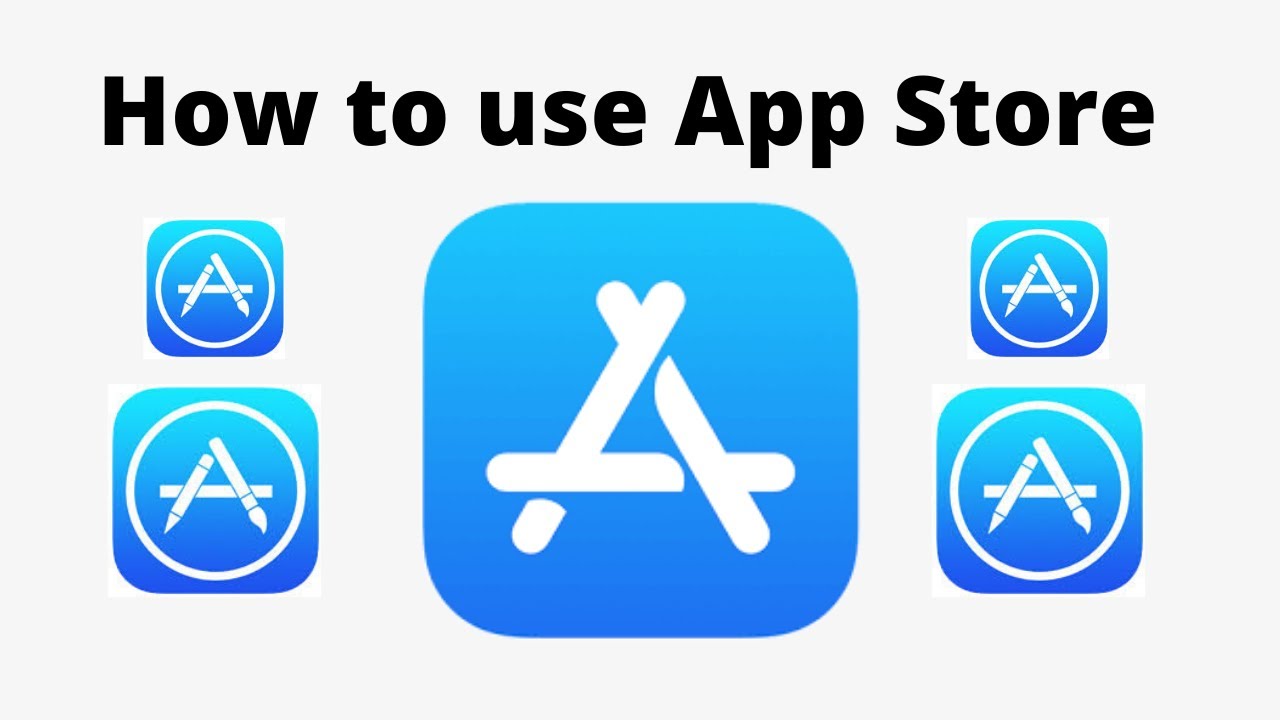The image features a minimalistic screen with a white background that showcases instructions on how to use the App Store in black text. Central to the composition is the prominent App Store icon, depicted as a blue rounded square with a stylized "A" composed of three overlapping lines. This main icon is flanked by two identical icons on each side, totaling to three pairs of stylized "A"s. The distinguishing feature of these icons is that the "A" on the left side has a pencil forming its left downward line, while the "A" on the right side incorporates a paintbrush for the right downward line. The arrangement creates a visually balanced and simplistic instructional image, with a total of five App Store logos arranged symmetrically around the central icon. The overall aesthetic is very clean and straightforward.